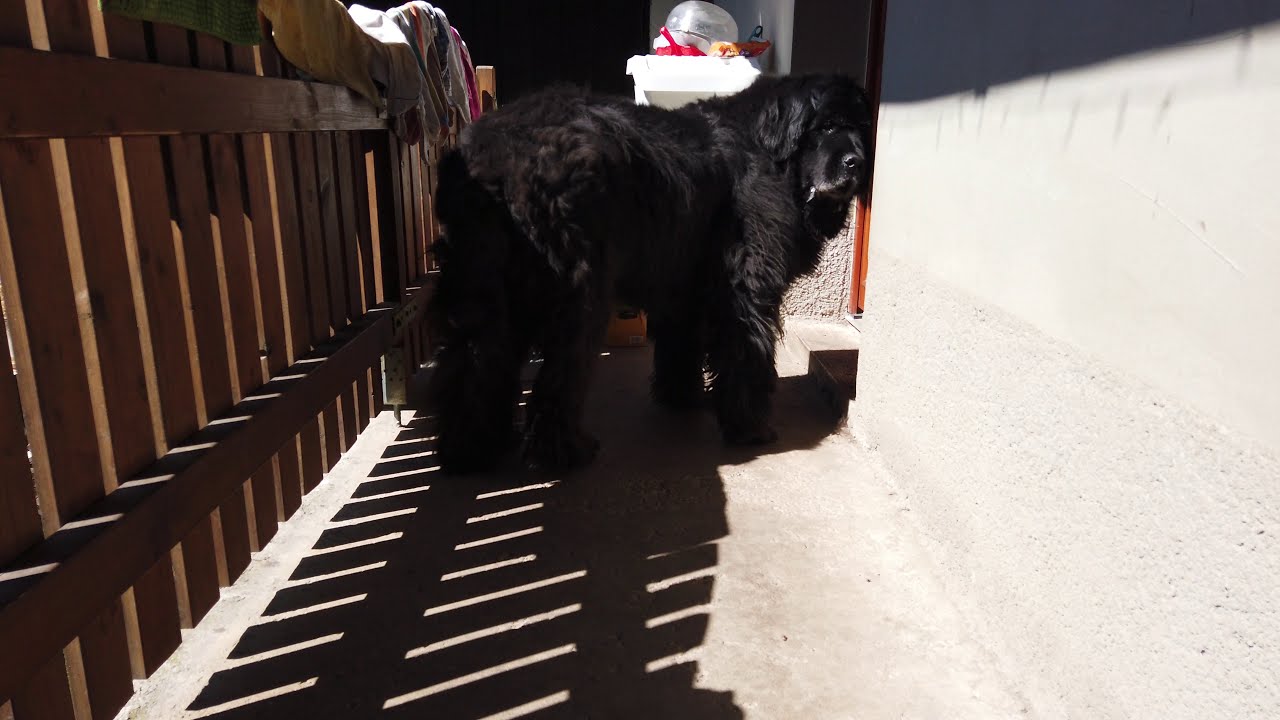The image features a narrow backyard or back balcony area with a gray cement patio extending from a doorway. A large, fluffy black dog reminiscent of a St. Bernard stands near the center of the patio, facing sideways with its body towards the doorway but its head turned back towards the viewer. Surrounding the dog is a sturdy timber fence made from thick brown wooden planks. Various articles of clothing and towels are draped over this fence, suggesting they have been hand-washed and laid out to dry. Behind the dog, near the wall, are tables and other stacked objects. The gray stucco building and the patio cast shadows that add depth to the scene. The photograph, in landscape orientation, provides a detailed and realistic glimpse of this quiet, homely setting.